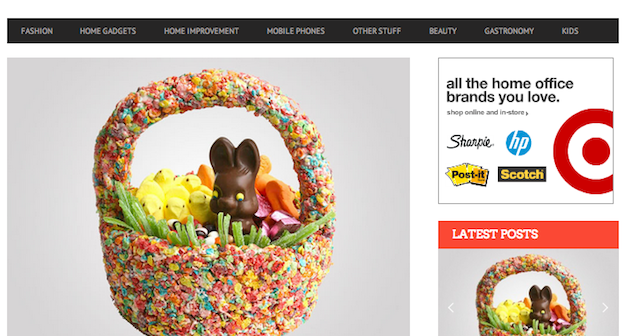The webpage likely belongs to a shopping platform with a design reminiscent of Target's, given the presence of the Target logo. The top navigation bar is black and contains categories in gray text, including Fashion, Home Gadgets, Home Improvement, Mobile Phones, Other Stuff, Beauty, Gastronomy, and Kids.

On the left side of the page, there is a vibrant Easter basket filled with Peeps and a chocolate bunny. What makes this basket unique is that it is covered in multicolored sprinkles, typically used for decorating cakes, adding a whimsical touch to the handle and the basket itself.

On the right, there is a promotional message that reads, "All the home office brands you love, shop online and in stores," featuring logos of popular office brands like Sharpie, HP, Post-it, and Scotch, accompanied by the Target logo.

Below this, the "Latest Posts" section displays the same Easter basket once more. This section accentuates the basket's lively color scheme, which includes hues such as orange, yellow, blue, green, brown, red, white, black, gray, and pink.